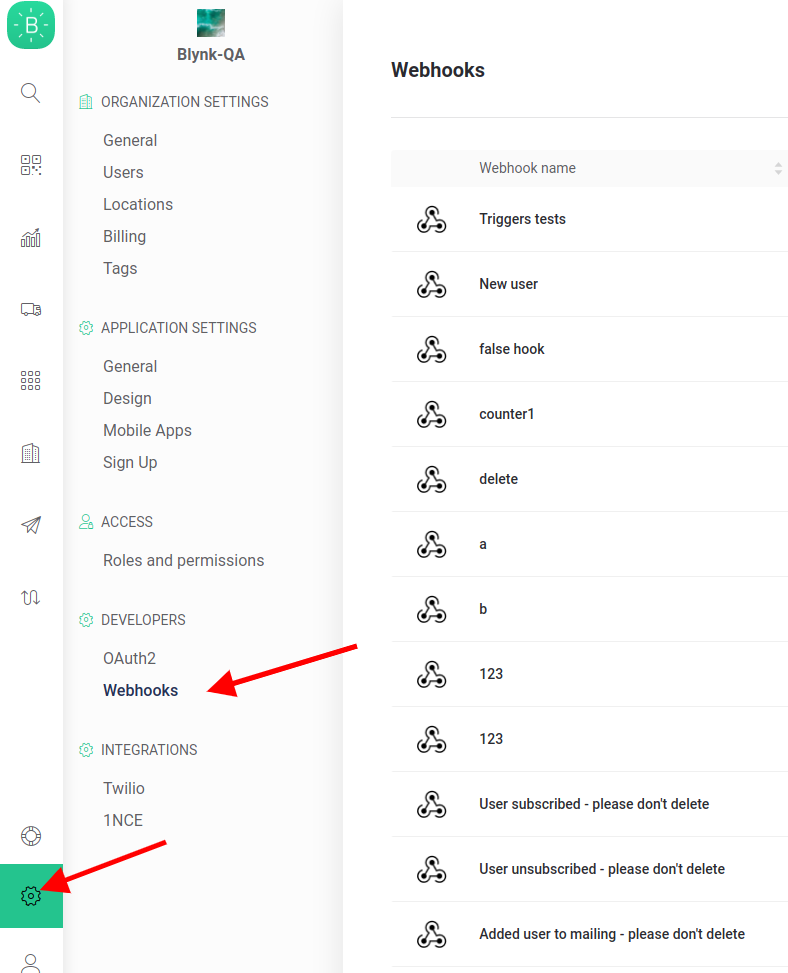The image presents a structured layout with a white background, featuring three distinct columns. 

The first column contains several icons and graphical elements. At the top, there is a small green square with a white letter "B," emitting small lines outward. Below this, there is a search button, followed by a series of other icons, including an 'Exit' symbol, a letter "M," a truck, a grid of nine dots, a building, an hourglass, and a sideways "S."

The second column showcases a block with a green picture and the title "Blink QA." This section is divided into several categories:
1. **Organizational Settings**:
   - General
   - Users
   - Locations
   - Billing
   - Tags
2. **Application Settings**:
   - General
   - Design
   - Mobile Apps
   - Sign Up
3. **Access**:
   - Roles and Permissions
4. **Developers**:
   - Zero off two

A red arrow points to the bold label "Webhooks" under the Developer section. Additional categories in this column include:
   - Integrations
   - Twila
   - One NCE

Another red arrow points to the left, indicating a green block labeled "Your Settings."

The third column focuses on details related to "Webhooks." This section lists various attributes and statuses:
- Webhook's Name
- Trigger Tests
- New User
- False Hook
- Counter 1
- Delete A
- B
- 1, 2, 3
- User Subscribe (annotated with "please don't delete")
- User Unsubscribe (annotated with "please don't delete")
- Added User to Mailing (annotated with "please don't delete")